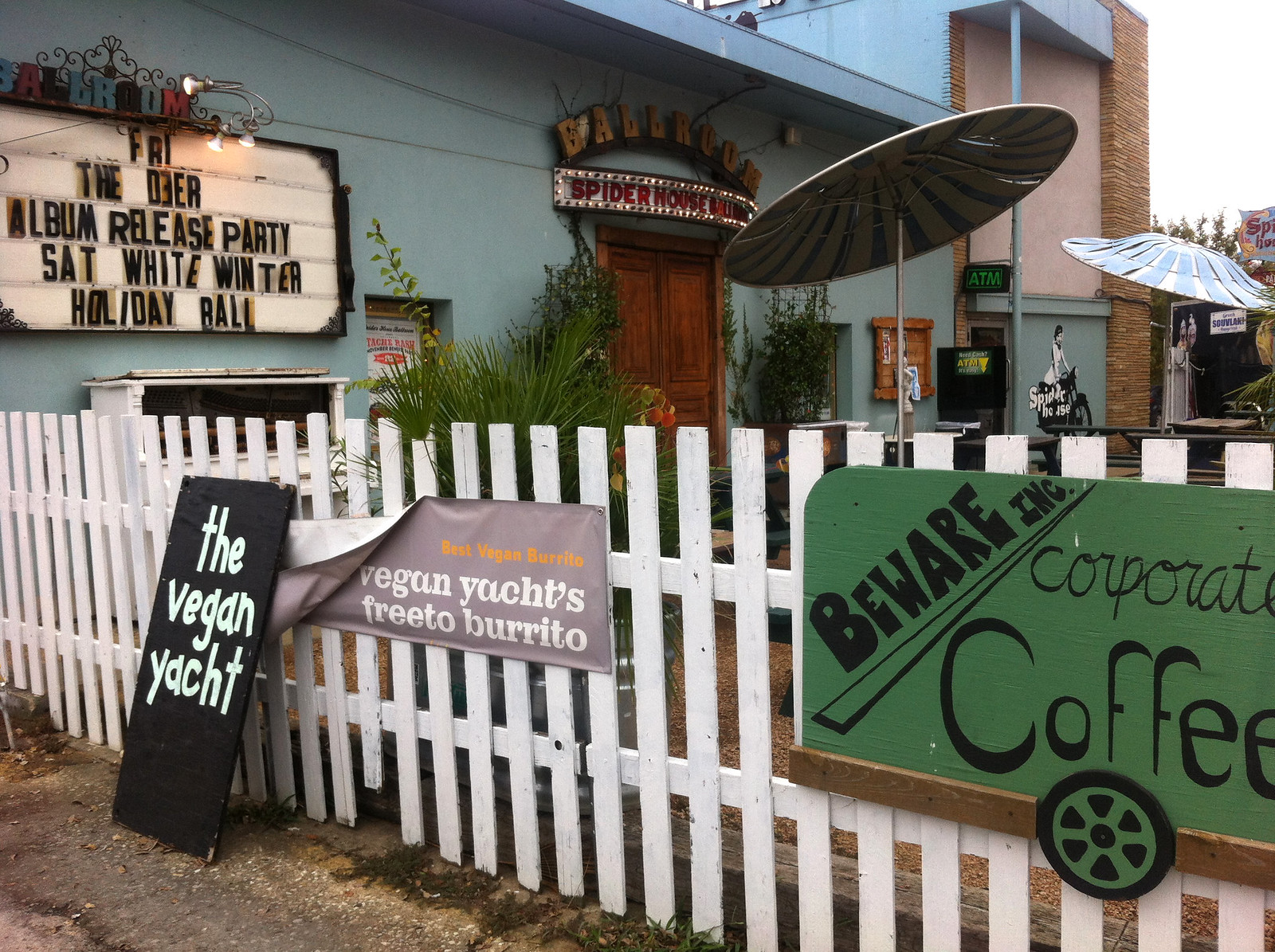The image depicts an outdoor setting in the middle of the day, likely just outside a combined restaurant and entertainment venue. The ground is covered by what appears to be a weathered stone walkway. In the foreground, there is a white picket fence adorned with several handwritten signs, which include phrases like "The Vegan Yacht," "Frito Burrito Beware, Inc. Corporate Coffee," and "Vegan Yacht Frito Burrito."

The centerpiece of the image is a building with a flat, bluish-gray roof, positioned centrally within the frame. On its wall, a billboard advertises events such as "Friday the 3rd Album Release Party" and "Saturday White Winter Holiday Ball." Above the entrance to this building is another sign, suggesting that it might be called "Spider House Ballroom."

Inside the fenced area, there are tables with umbrellas, indicating a seating area for the patrons. The scene is enriched with a variety of colors including gray, black, white, purple, orange, green, and tan. The overall ambiance suggests that this establishment serves as a communal space featuring both dining and entertainment options, possibly doubling as a restaurant and ballroom.